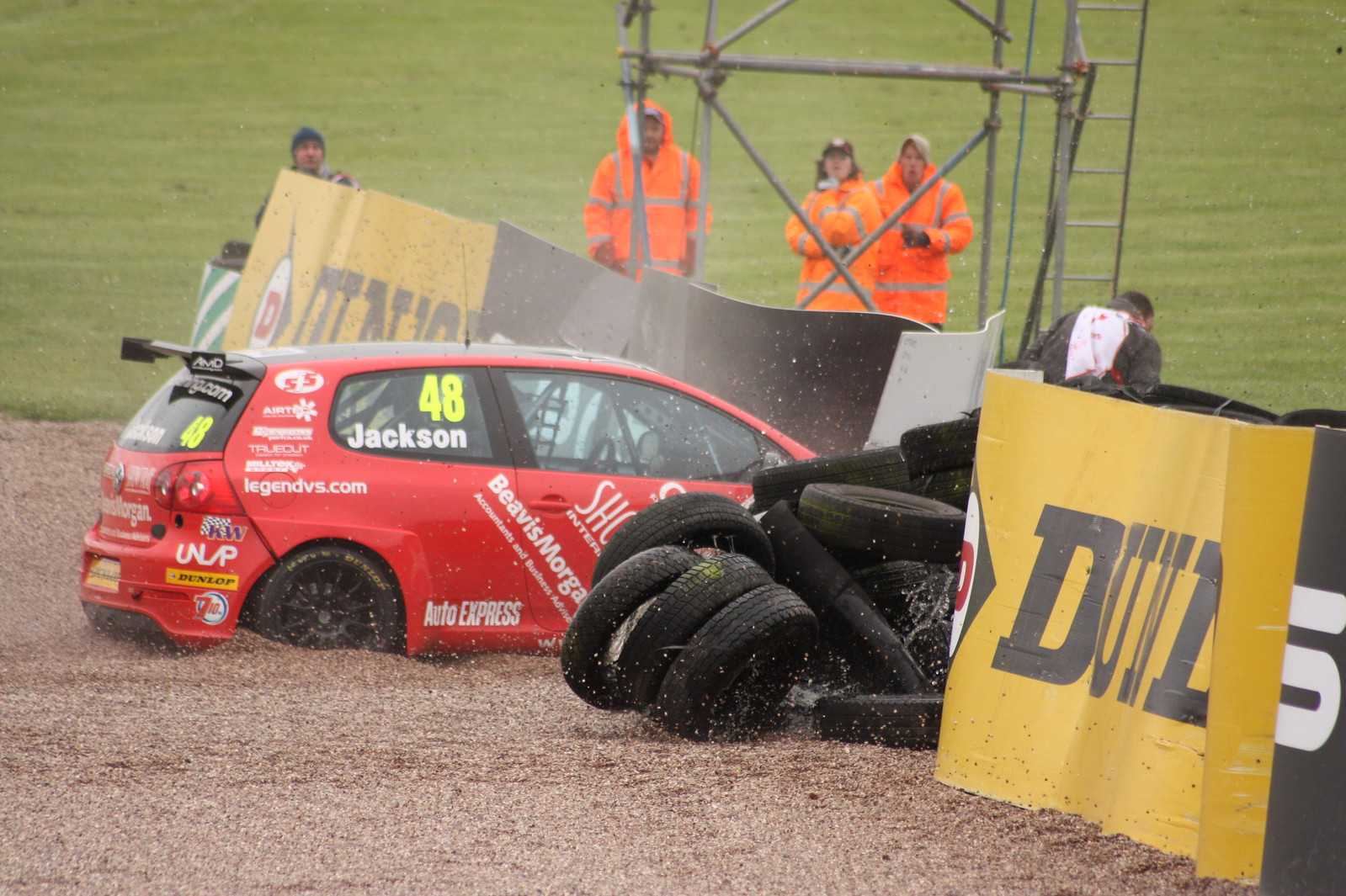In this image, we see an outdoor setting, likely in the middle of the day at a demolition derby or rally event, with various textures and elements. The scene starts at the bottom with a muddy or sandy surface transitioning to a grassy texture at the top. Central to the image is a red car, resembling a VW Golf, adorned with numerous decals and stickers, including the number 48 and the name "Jackson" on the back quarter panel window. This car appears to have spun off the road and is crashing into a pile of tires, surrounded by gravel and flying debris. Next to the car is a stack of ladders, and a dividing wall runs parallel to the scene. On the far side of the wall, several crew members or emergency staff wearing orange hi-vis jackets can be seen standing and observing the scene. The colors in the image prominently include brown, yellow, black, white, orange, gray, and green, contributing to the detailed and chaotic atmosphere of the event.